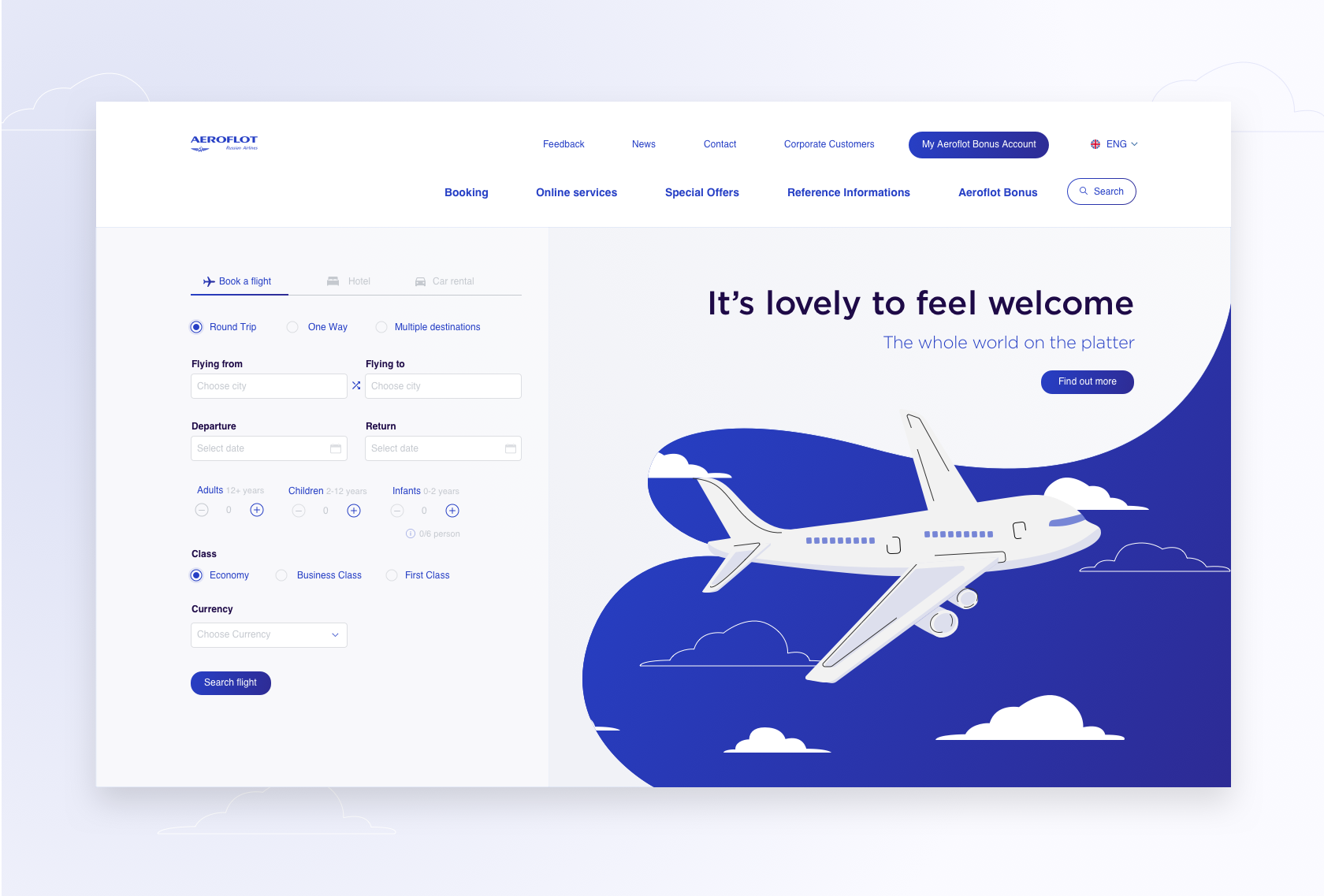The image portrays a computer screen with the Aeroflot website open. The website prominently features the Aeroflot logo accompanied by wing graphics. The navigation bar includes various drop-down menus labeled: Booking, Online Services, Special Offers, Reference Information, and Aeroflot Bonus. At the top, smaller options are available for Feedback, News, Contact, Corporate Customers, and My Aeroflot Bonus Account. Users have the option to view the site in English or another language.

On the right-hand side of the screen, there is an image of a white airplane with blue windows, soaring through a royal blue sky dotted with white clouds and some clouds with blue centers and white outlines. The text overlaying the image reads, "It's lovely to feel welcome," followed by the phrase, "The whole world on the platter," and a "Find Out More" button.

The left side of the image features the booking section, where fields are provided for entering details such as departure and destination points, departure and return dates, number of adults, children, infants, travel class preferences, and currency selection.